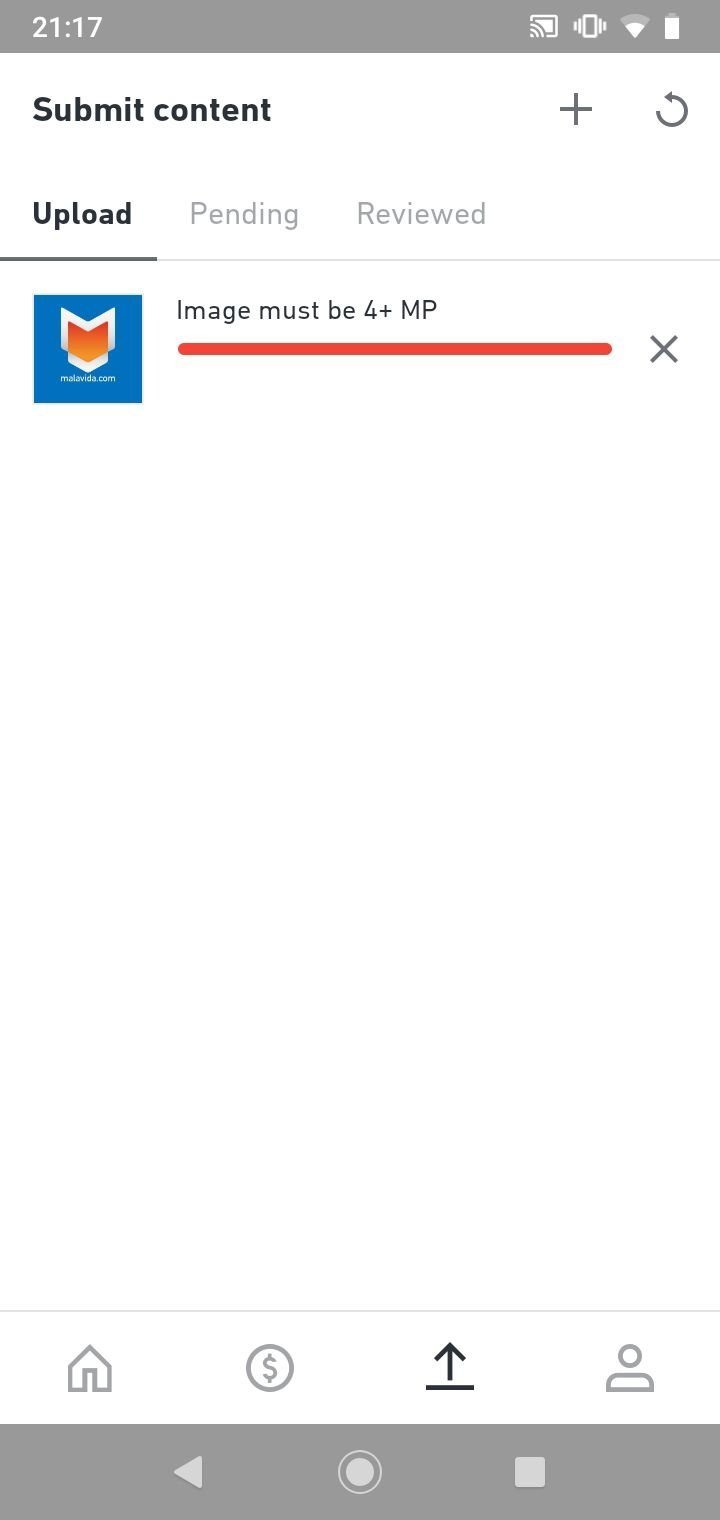This screenshot appears to be taken from a cell phone. At the top of the screen, within a gray text box, the time is prominently displayed as 21:17 alongside traditional status icons for web connection, signal bars, and battery life. 

Below the time and icons, in bold black letters on a white background, the text "Submit Content" is clearly visible. Adjacent to this text is a plus sign for adding new content and a circular refresh icon.

The next section offers three clickable options labeled "Upload," "Pending," and "Reviewed" meant for managing content status. 

On the left-hand side, there is a blue box with an orange chevron-like design in the center. This box is accompanied by a red status bar, signaling a critical status alert which states, "Image must be 4+ MP" with an 'X' icon for canceling the message.

At the bottom of the screen, from left to right, there are multiple interactive buttons: a home button, a dollar sign (potentially for cashing out), an upward arrow for uploading, an icon depicting a user's profile, a left-facing triangle for navigating back, a central button likely for starting or stopping actions, and a square stop button on the right.